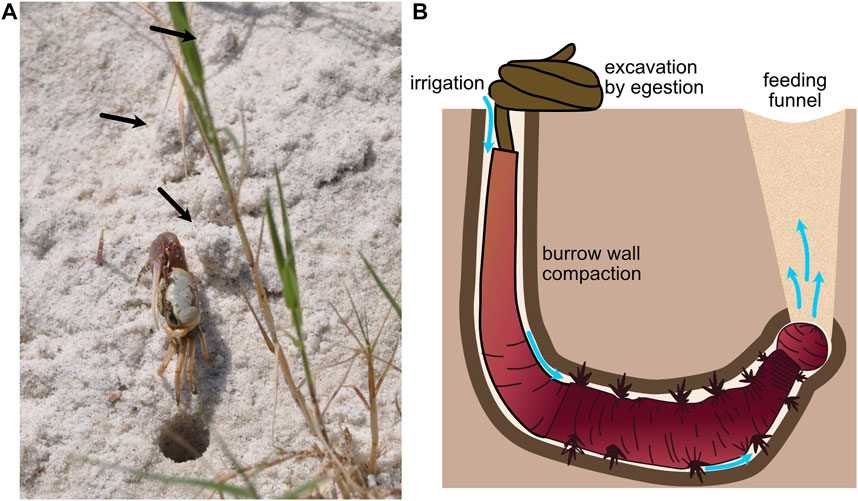This image consists of two distinct parts: 

On the left-hand side (labeled A), there is a vertical rectangular photograph of a light-colored crab walking on white sand. The sandy beach also features a few blades of beige and green grass sprouting from it. A small hole is visible in the sand, located slightly below the crab. Above the crab, three black arrows point to various parts of the sand, indicating specific areas of interest.

On the right-hand side (labeled B), there is a detailed illustration, presumably linked to the crab's habitat. The illustration depicts a red worm-like creature with about ten black legs burrowing through the sand. It showcases the process of excavation by egestion, where the worm consumes soil and expels waste, forming a trail behind it. The illustration includes several labels, such as "burrow wall compaction," "irrigation," and "feeding funnel," with blue arrows indicating the direction of the worm's burrowing path. The winding intestine-like structure emphasizes the creature's movement and the compaction of its burrow walls.